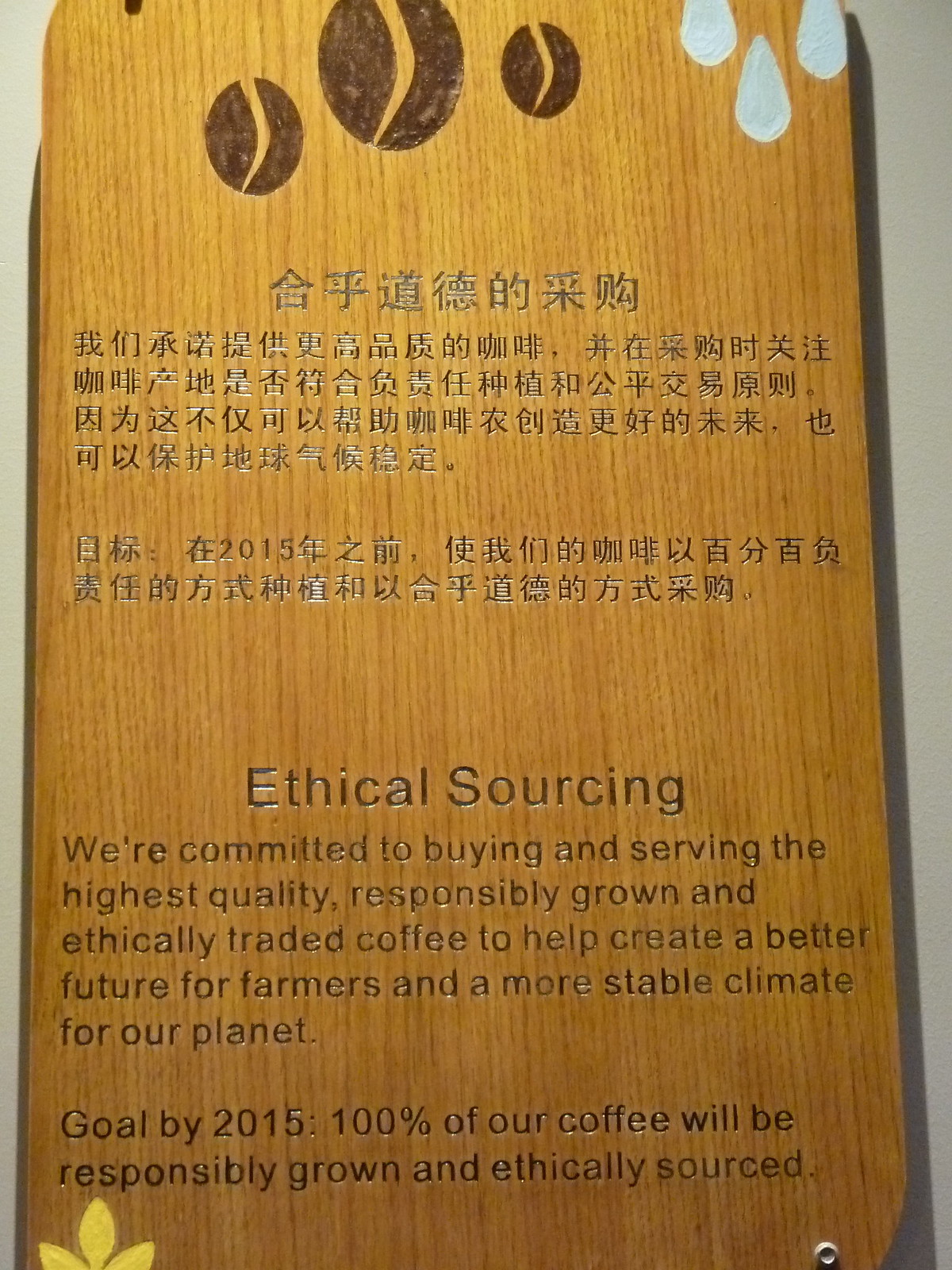The image features a vertically oriented, rectangular wooden sign mounted on a gray wall. The sign's background is brown, and it prominently displays an ethical sourcing message in both Chinese and English. At the top, there are illustrations of three coffee beans and three white teardrop-shaped symbols. Below these illustrations, the text "ethical sourcing" appears, followed by a detailed commitment: "We're committed to buying and serving the highest quality, responsibly grown, and ethically traded coffee to help create a better future for farmers and a more stable climate for our planet." Further down, it states their 2015 goal: "100% of our coffee will be responsibly grown and ethically sourced." The sign also features a yellow flower at the bottom left and a screw in the bottom right, which secures it to the wall.